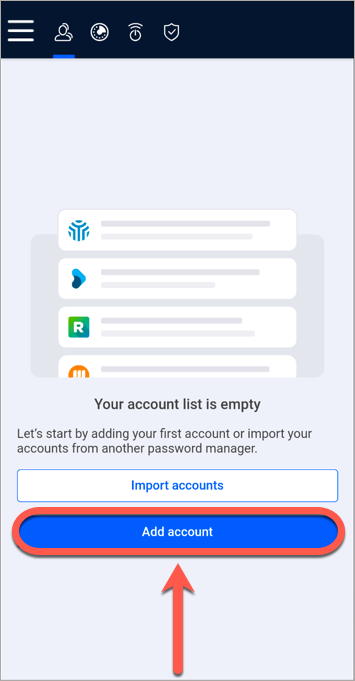This image is a mobile phone screenshot that has been turned into a tutorial. The background of the screen is pale gray. At the top, there is a black bar containing multiple icons in white: three parallel horizontal lines on the left, followed by two line drawings of people, a circle with a pen-like symbol inside, a clock with two lines above it, and a shield with a tick mark. 

Below this black bar, the pale gray background continues. A blue underline highlights the icon representing the user account, indicating the current section being viewed.

In the center of the screen, there is a darker gray box with at least four white rectangular boxes layered on top of it. Each box features distinct symbols: the first box contains a circle with blue lines, the second shows a blue arrow pointing right, the third is a green square with an 'R' in white, and the partially obscured fourth box features an orange circle with a 'W'.

A light gray pop-up message is displayed in the center of the screen, stating "Your account list is empty. Let's start by adding your first account or import your accounts from another password manager." Below this message, there is a white button outlined in light blue with the text "Import accounts" in blue, and underneath that is a blue, capsule-shaped button with "Add account" written in white.

To draw attention to the "Add account" button, it has been outlined with a thick red line, and a large, thick red arrow points upwards towards it from the bottom center of the image.